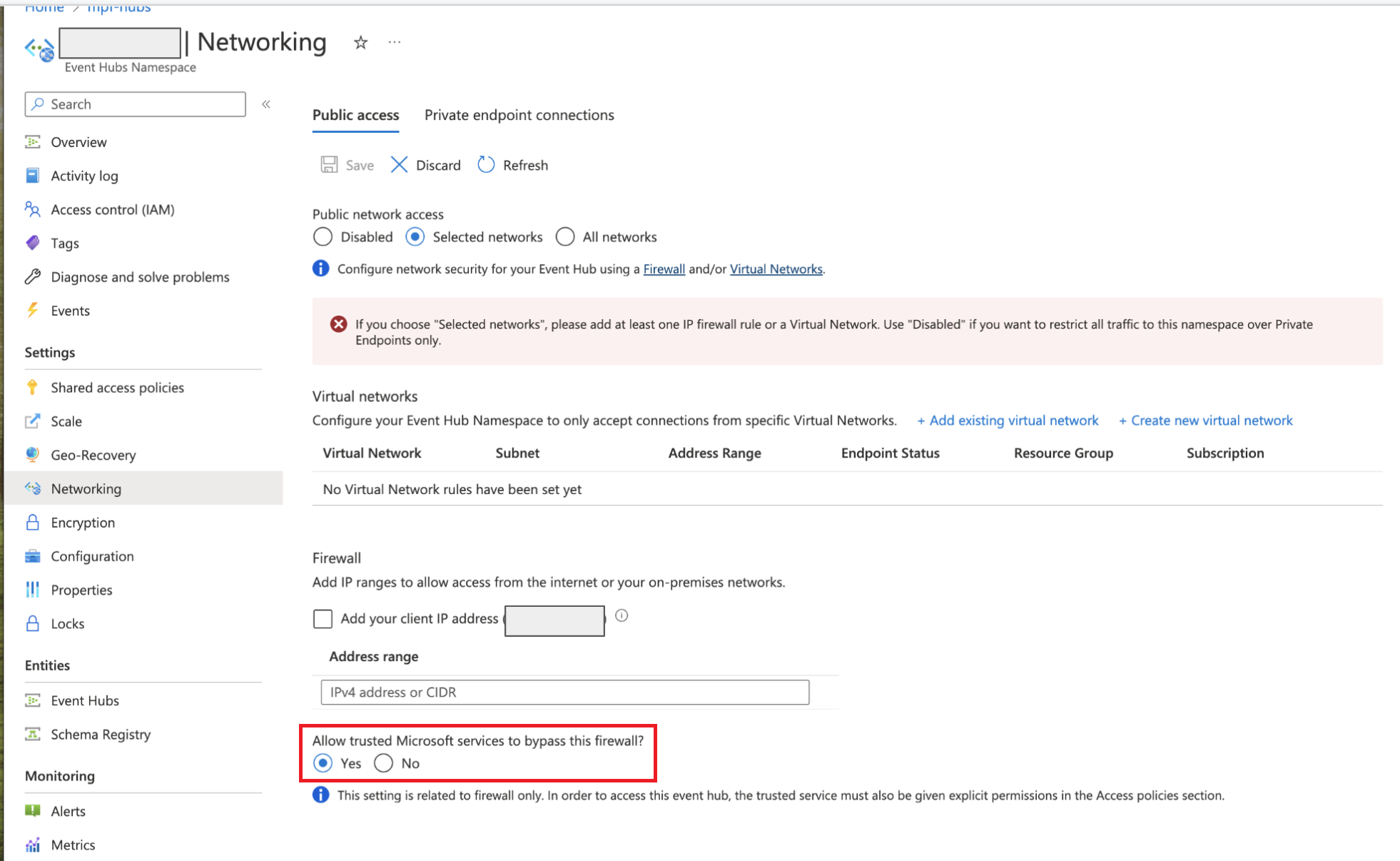A screenshot from an IT network settings page on a website resembling a Windows computer interface. The page has a white background with dense black text and blue elements detailing various technical aspects. It covers categories such as networking, geo-recovery, encryption, schema, registry, event hubs, activity log, and access control. The user currently navigates the Networking section, specifically the Public Access subsection. The settings involve configuring a firewall, with the option to allow trusted Microsoft services to bypass it highlighted in a boxed area at the bottom. This setup appears incomplete, indicating the page is in the process of being configured for a complex business network by IT professionals.